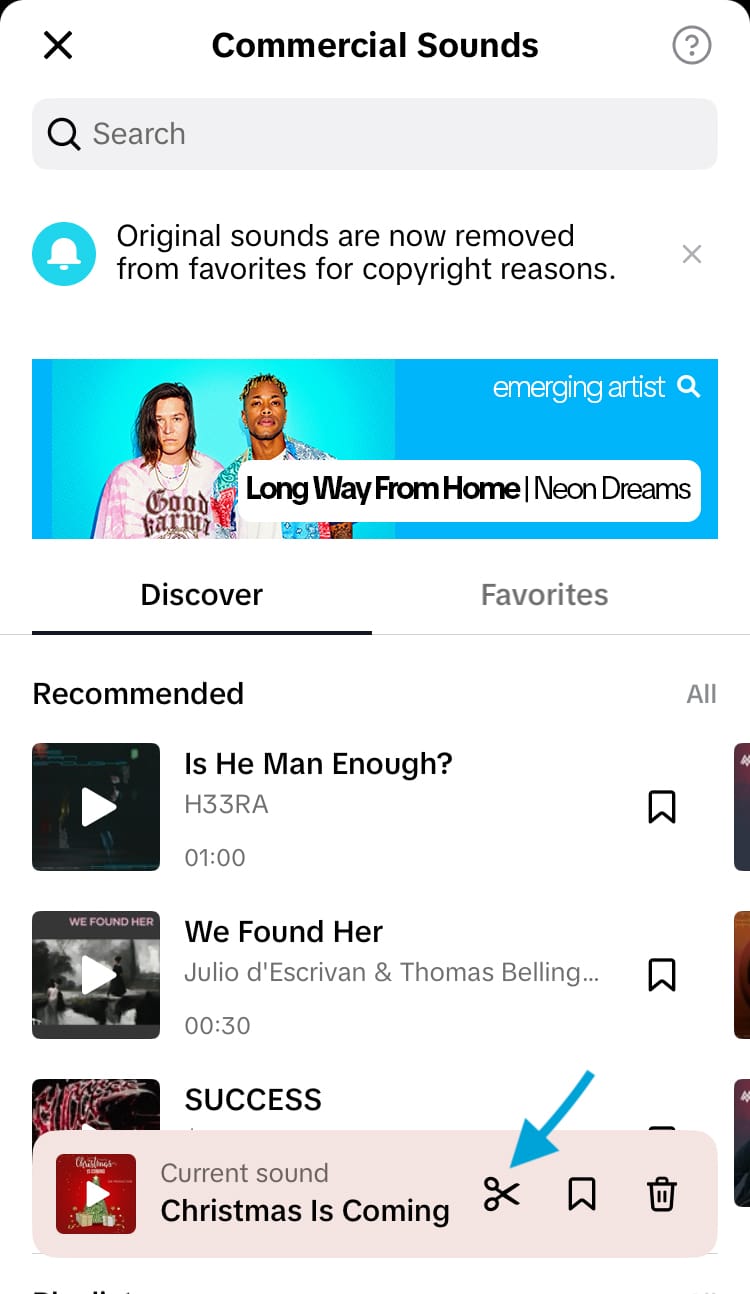The image is a screenshot from a smartphone displaying a specific section titled "Commercial Sounds." At the top of the image, a notification reads, "Original sounds are now removed from favorites for copyright reasons."

Beneath this message, there is a teal-colored area featuring a photograph of a couple. The woman, a Caucasian, wears a "Good Karma" shirt and has a serious, almost mug shot-like expression. Next to her stands an African American man who has a neutral expression. Accompanying this image is the text: "Long Way from Home" and "Neon Dreams," followed by "Emerging Artist."

As we scroll down further, the interface shows options for "Discover" and "Favorites," with "Discover" currently selected. Below this, there is a section labeled "Recommended." Here, song titles such as "Is He Man Enough," "We Found Her," and "Success" are listed. However, "Success" is partially obscured by a label reading "Current Sound."

Additionally, there is a teal-colored arrow pointing towards a pair of scissors icon, suggesting an option to cut the song if it is not preferred. A trash button is also visible at the end, likely for deleting the song. In the middle section, a ribbon icon is displayed, though its exact purpose is not specified.